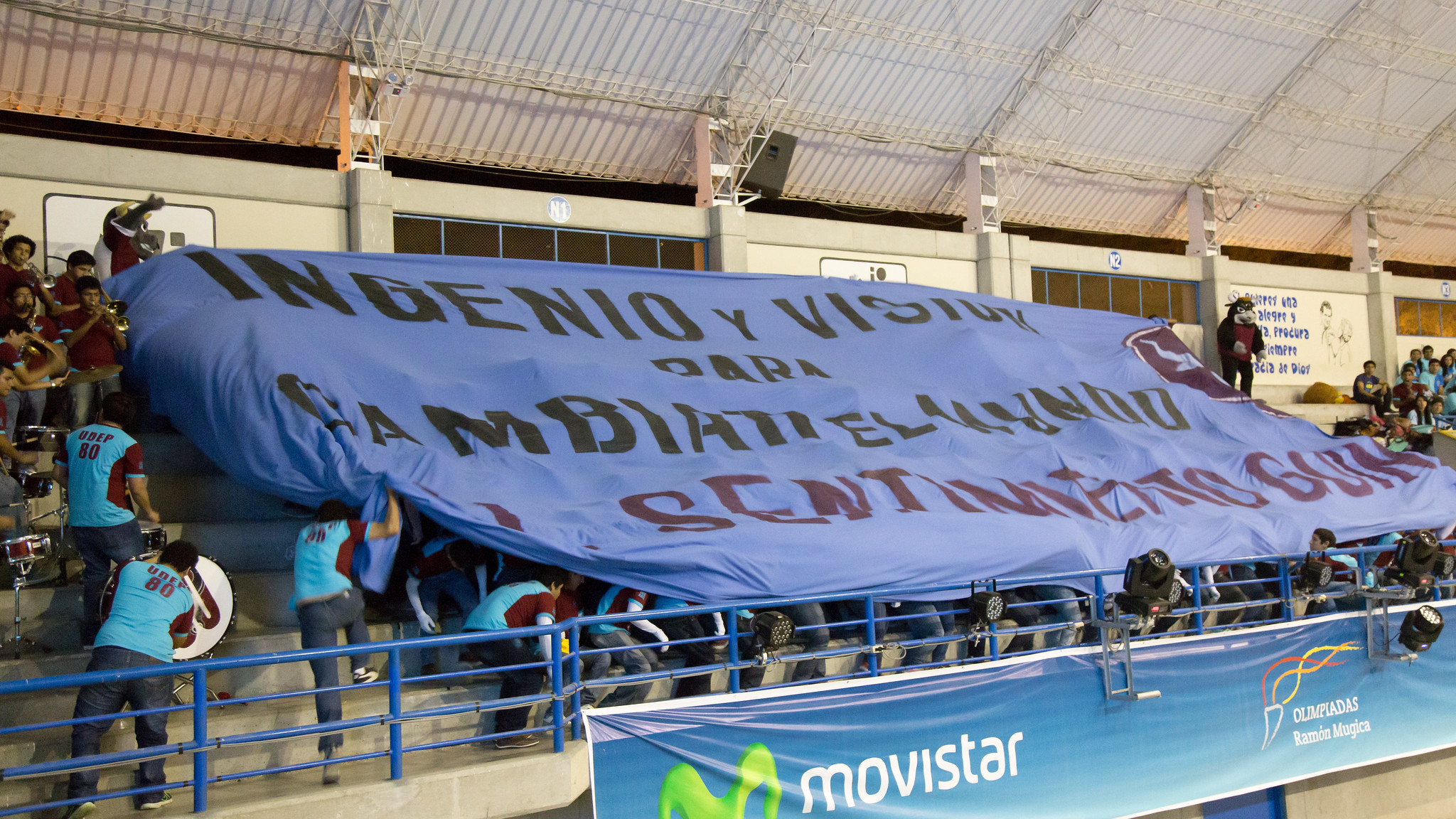The image captures an indoor stadium scene predominantly featuring the colors white and blue. It showcases a crowd of spectators seated in bleacher-like stands, partaking in what appears to be a soccer or football match. The stadium is adorned with several banners, one of which reads, "Ingenio e Visto para Dambiente Centenario," along with another banner displaying "Movistar" with a green 'M' symbol. Additionally, there's a vibrant sign that says, "Olimpidades Racion Majada," featuring red and yellow intertwining symbols. To the left side of these signs, there is a group of children, possibly of Indian origin, dressed in white and blue shirts with maroon sleeves, playing musical instruments like saxophones and trumpets. The stands are also draped with a massive blue cloth banner with black Spanish text, which the audience members are holding up. The scene is lively and colorful, combining elements of a sports match with celebratory performances.